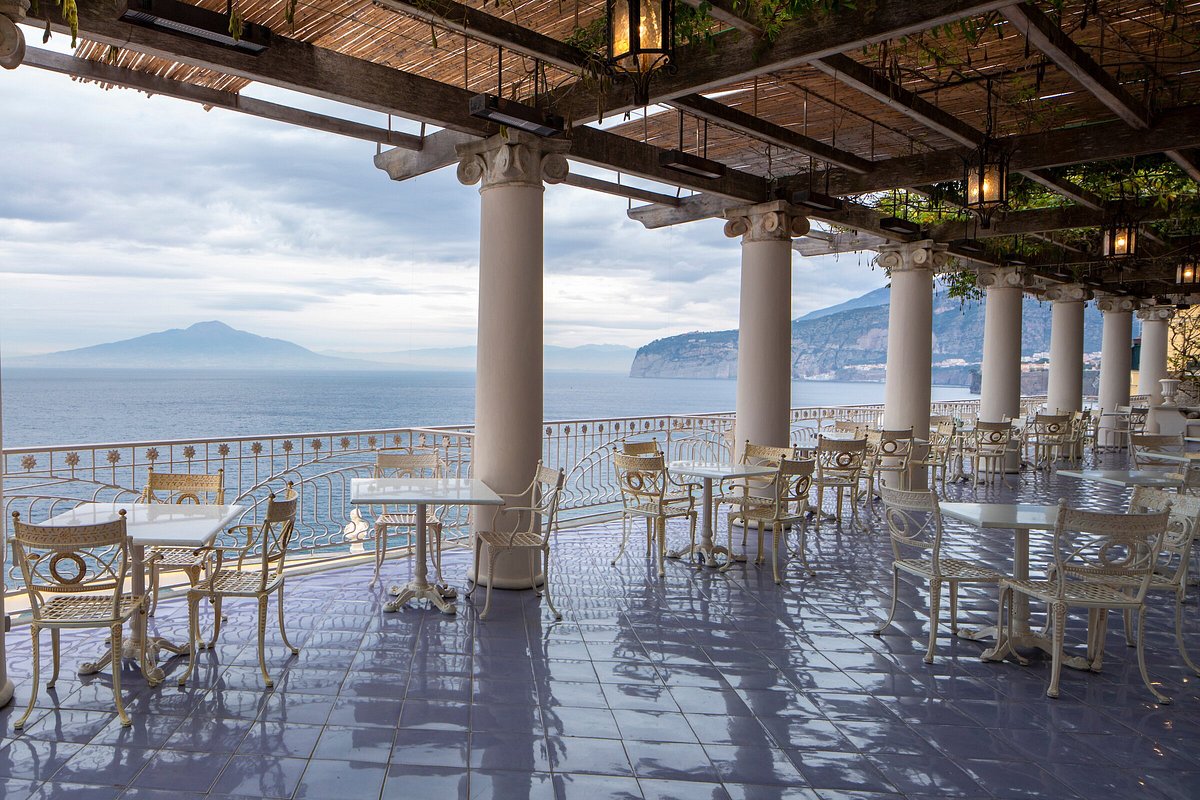The image showcases a beautifully designed outdoor seating area of what appears to be an upscale restaurant or reception hall situated by a body of water. The foreground features a shiny gray floor that almost looks wet, perhaps from recent rain, with about twenty ornate, vintage white cast-iron tables and chairs, each topped with square white surfaces supported by pedestals. This setting is under a brown pergola-style roof supported by elegant white pillars, adorned with lanterns hanging from the ceiling, adding to the vintage charm. Above portions of the roof, straw-like materials and greenery can be seen, contributing to a natural, resort-like ambiance.

In the background, beyond a white railing, one can see a vast waterway, with hazy mountains and landmasses dimly visible under a cloudy daylight sky. One triangular landmass stands prominently in the distance, while another, slightly darker landmass rises above the right side of the ceiling structure. The setting is well-lit despite the cloudy weather, enhancing its tranquil and picturesque quality. Although the scene is devoid of people, it exudes a serene and inviting atmosphere, perfect for dining with a stunning view of the ocean.